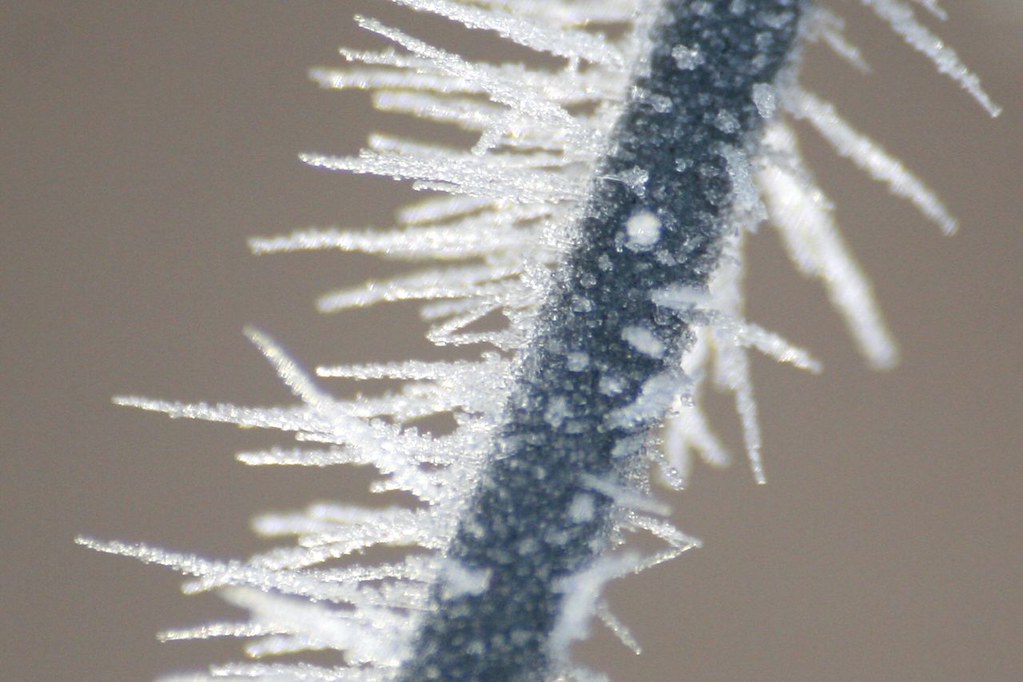This photograph, set against a blurred light beige background, captures a close-up view of a thin, dark brown to borderline black branch or metallic rod positioned diagonally from the center to the top right of the image. Adorning the branch/rod are numerous white crystalline structures, which are likely composed of either ice or sugar. These structures extend outward in thin, straight, horizontal lines, creating a pointy and irregular texture across the surface. Each crystalline formation is unique, reflecting subtle differences in design and pattern while maintaining a general uniformity in size and shape. Despite the simplicity of the image, the abstract and detailed arrangement of the crystalline protuberances instills a sense of mystery and intricate beauty.